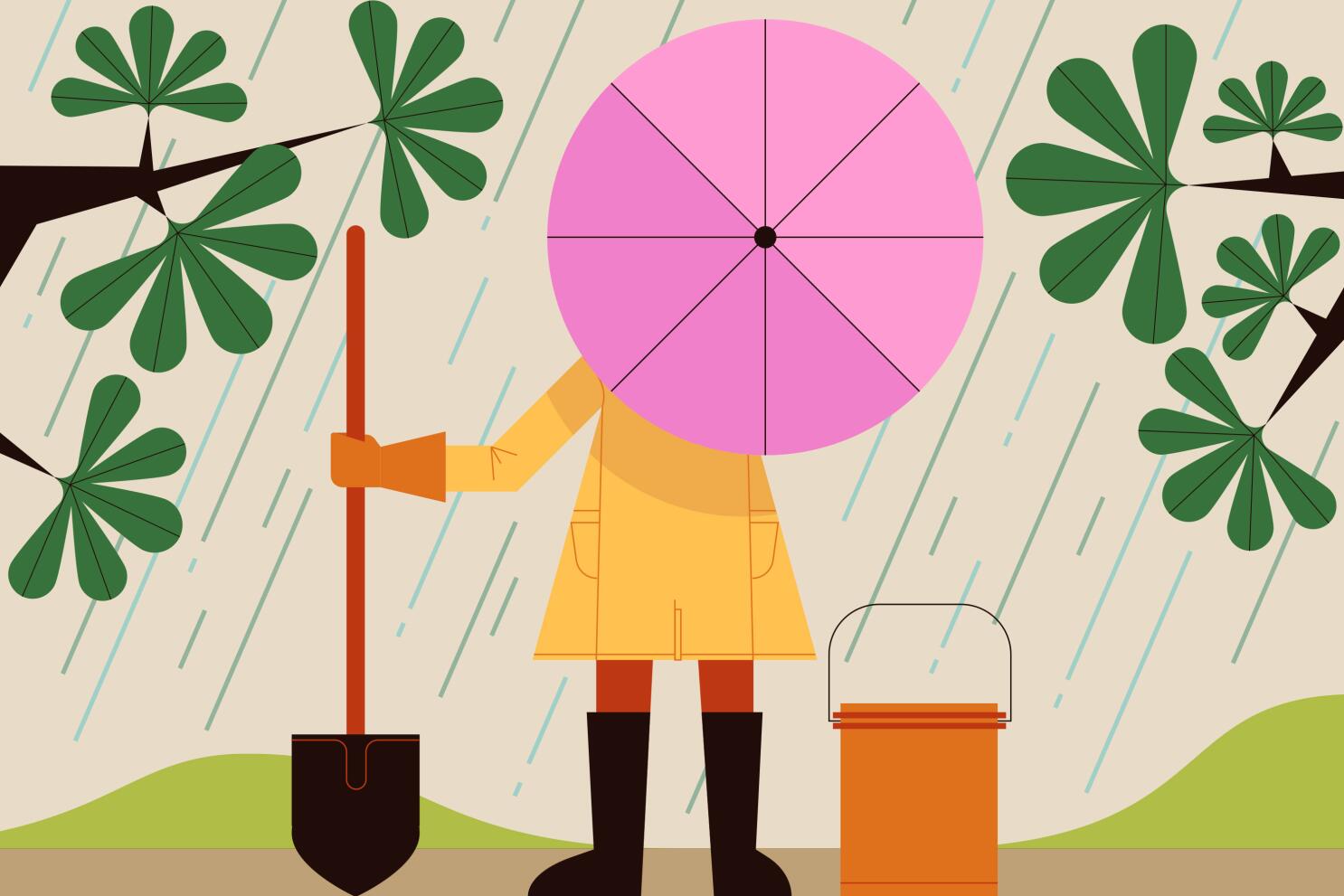The image is a cartoon-style drawing depicting an individual working in the yard on a rainy day. Standing on a light tan, dirt-like ground, the person is dressed in brown boots, orange pants, a yellow raincoat, and orange gloves. They are holding a pink umbrella with visible black support lines extended in front of their face, obscuring their head and one arm. In their right hand is a shovel with an orange handle and a brown spade. The background illustrates several green hills, streaks of green rain, and an off-white, rainy sky. To the left of the person, there is an orange bucket with a thin silver handle. Flanking the scene are dark brown tree branches with green, tear-shaped leaves; each branch contains five leaves. The overall color palette includes green, dark brown, tan, orange, pink, and off-white, creating a vivid and detailed representation of the rainy garden scene.